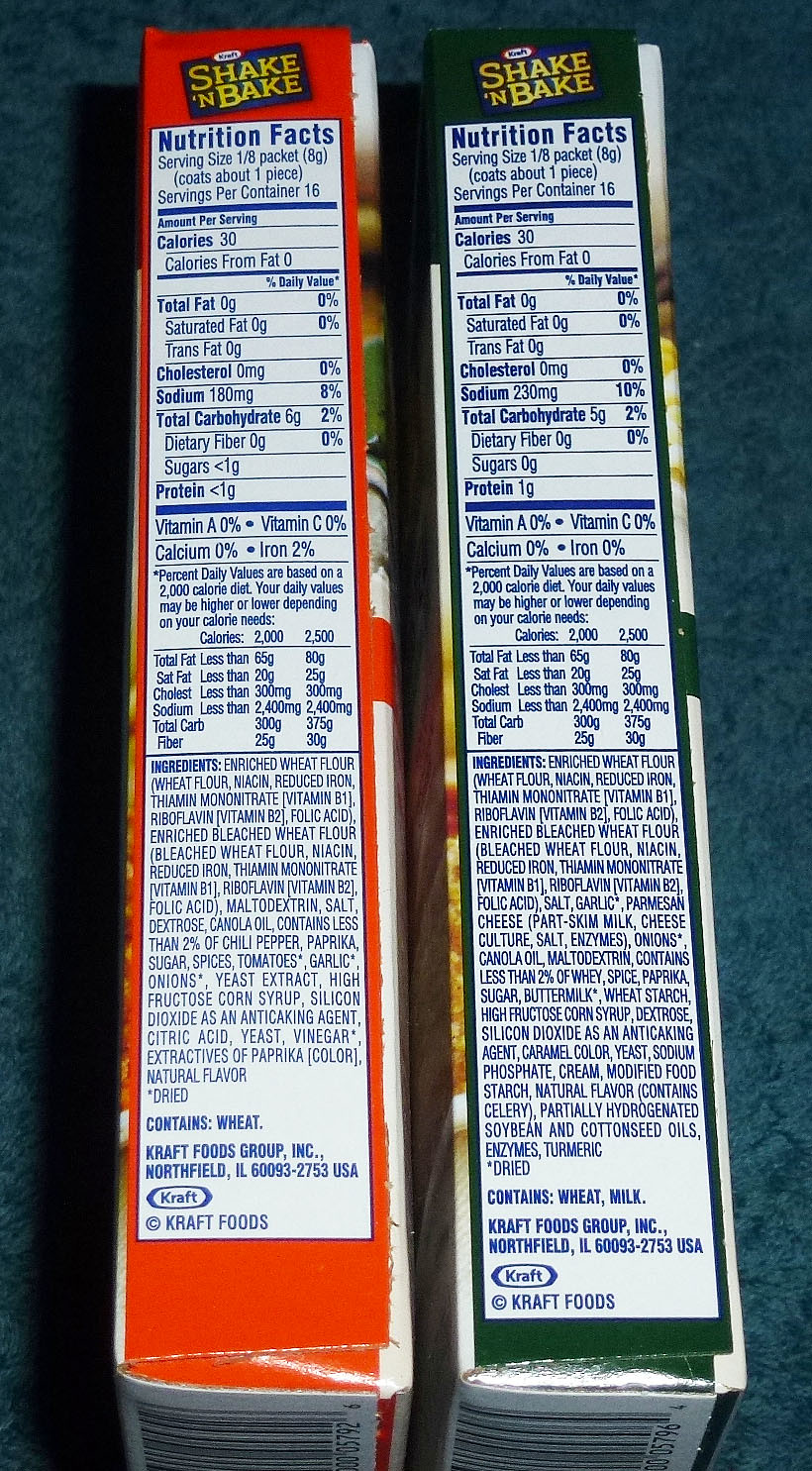The image depicts two vertically-aligned, side-by-side shake-and-bake boxes manufactured by Kraft Foods. The focus is on the nutrition facts and ingredients listed on the side flaps of each box. One box has a red outline, while the other has a black outline. Both boxes appear somewhat worn at the bottom edges and provide detailed nutritional information, listing total fat, calories, proteins, serving sizes, and specific ingredients down to warnings such as 'contains wheat.' The text indicates the product is made by Kraft Foods Group in Northfield, Illinois, USA. The background appears to be a low-pile blue carpet, evident from the small dents visible on its surface. This close-up shot is in portrait orientation, emphasizing the detailed comparison of the nutritional content between the two different-colored packages.